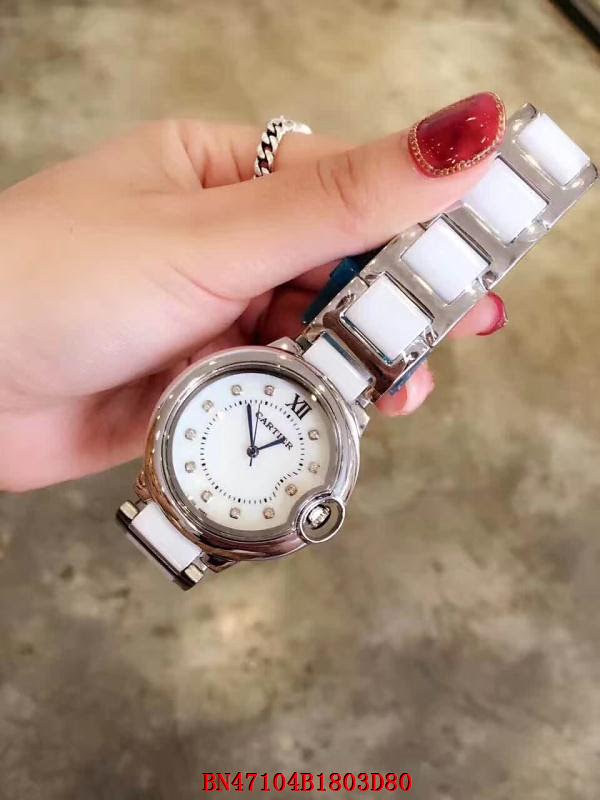In the photograph, a person's hand is prominently displayed against a blurry background that appears to be a gray floor, though it's unclear if it's cement or carpeted. The hand, coming from the left of the image towards the center, has shiny red painted fingernails and a silver braided ring on the pointer finger. The hand is holding a sophisticated Cartier watch with an entirely silver wristband. The clock face of the watch is white, featuring black hands and gold circular symbols in place of numbers, except for the top middle where the number 12 is marked in Roman numerals. Additionally, small diamonds seem to replace the usual numbers. At the bottom of the image, red text displays a watermark or code: BN47104B1803D80. The woman's skin tone is white, and the background also includes what seems to be a roughed-up, granite-like table with white and brown coloring.